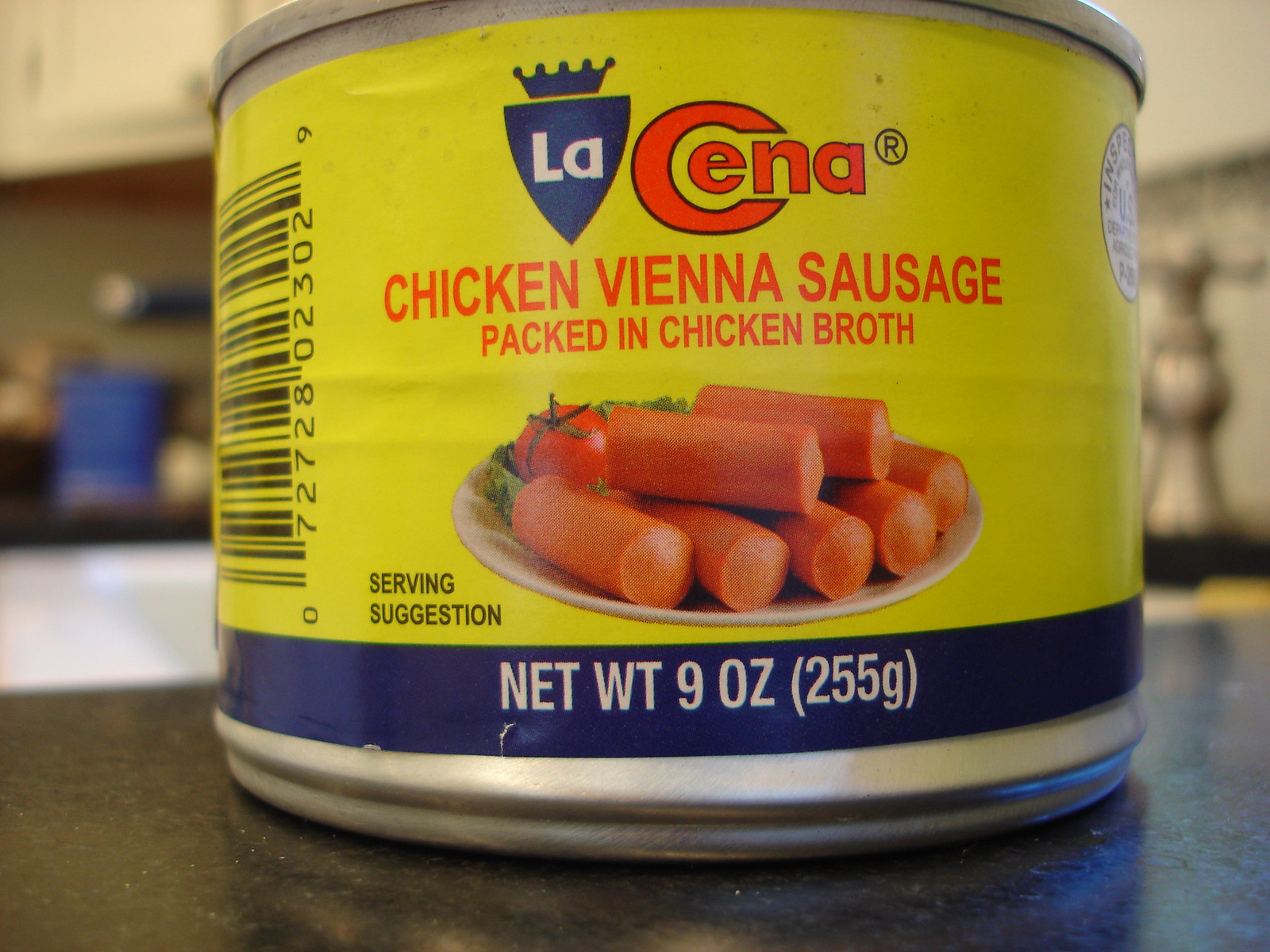The photograph captures a close-up image of a silver can of La Sina chicken Vienna sausage, packed in chicken broth, resting on a black countertop. The can features a predominantly yellow label with a dark blue band at the bottom. At the top of the label, "La Sina" is displayed in blue, with "chicken Vienna sausage packed in chicken broth" written beneath in red. The middle of the label showcases a serving suggestion, depicting a ceramic plate with five Vienna sausages neatly arranged at the bottom and two more angled artistically on top, accompanied by a piece of lettuce and a tomato. The label also notes the net weight as nine ounces (255 grams). Additionally, there's a black barcode on the left side of the label, numbered 0-7-2-7-2-8-0-2-3-0-2-9. In the top right, a white circle indicates the product has been inspected by the U.S. Department of Agriculture. The background reveals a slightly out-of-focus kitchen with white cabinets and a faucet handle to the right, suggesting the can is placed near a sink.